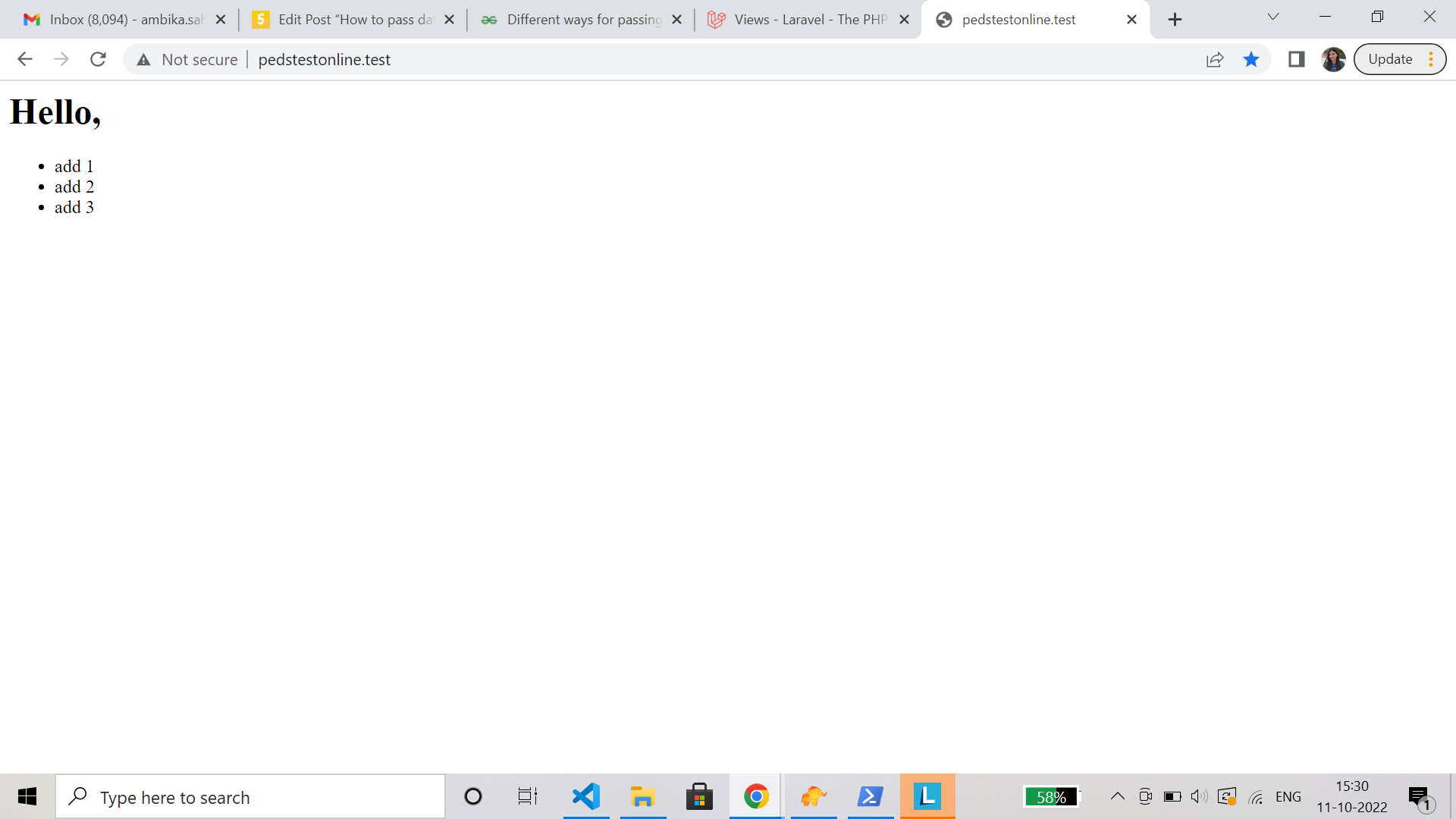The browser window displays five open tabs, with the current active tab labeled "PEDS TEST ONLINE.test." The website's address, visible in the URL bar, reads "PEDS TEST ONLINE.test" and is marked as not secure. The webpage is mostly blank, featuring a minimalist design with only a greeting in the upper left corner that says "hello," followed by three bullet points labeled "Add one," "Add two," and "Add three."

In the background, the other open tabs reveal a clutter of activities: an inbox with an overwhelming number of unread emails, indicated as 8,094, a tab titled "Edit Post," another fading tab concerned with passing exams or skills, and a partially visible tab related to learning "LARAVEL - the PHP."

At the bottom of the screen, various icons are displayed, though their specific functions remain unclear. One recognizable icon is a file, hinting at possible document management or downloads. The overall scene indicates a busy and somewhat disorganized browsing session.